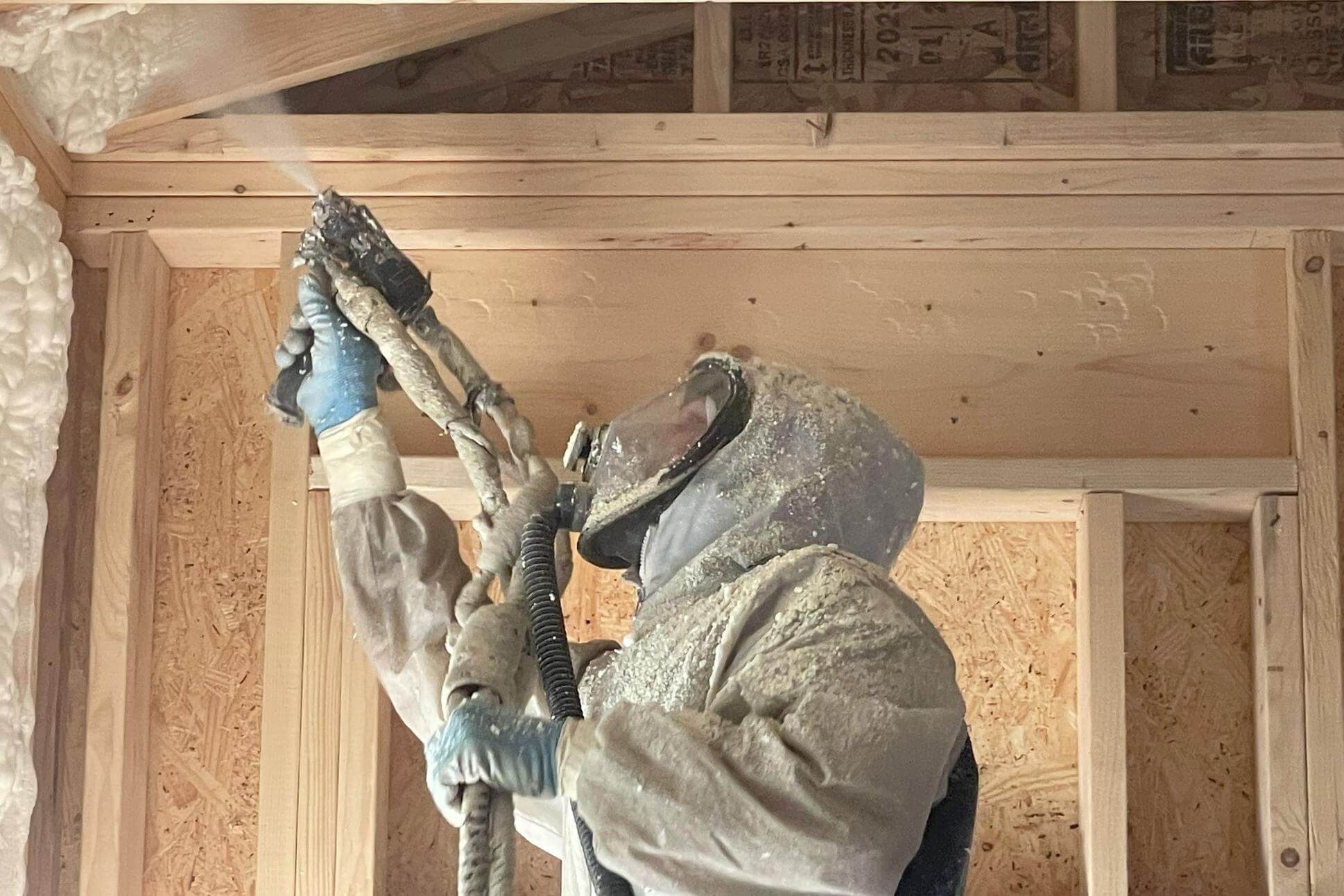The image depicts a professional insulator at work inside an unfinished home, likely in the attic or upper level. The construction site reveals the raw wooden framework of the house, characterized by light beige and light brown hues. There are no drywall panels installed yet, showcasing only the structural beams and plywood boards. The worker, facing left, is meticulously applying foam insulation to the corners and rafters using a specialized spray gun connected to gray hoses. His protective gear includes a full-body gray suit covered in foam residue, blue gloves taped at the sleeves for added protection, and a mask akin to a gas mask to ensure safety while handling the insulation materials. The site is visibly filled with construction dust, further underscoring the ongoing building efforts. This careful insulation work hints at the future placement of a door behind him, though the primary focus is on the accurate and thorough application of the foam.